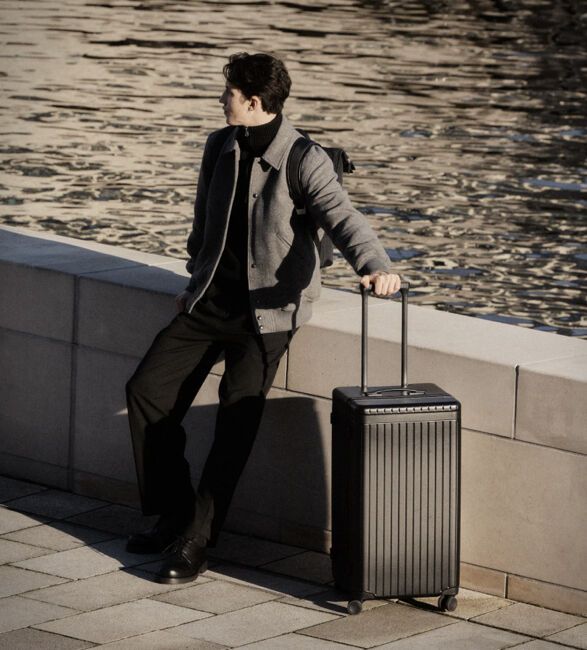In this photograph, a dark-haired man is leaning against a short white stone wall near a body of water, which could be a river or lake. He's wearing a gray overcoat over a black turtleneck or shirt, paired with black pants and black shoes. The man has a backpack indicated by a visible nylon strap over his shoulder, and he's also holding the handle of a tall, rectangular black suitcase with four wheels. The handle of the suitcase is extended upwards. The water behind him is rippling and glistening under the sunlight, suggesting a bright day. He is standing on a gray-tiled sidewalk, looking off to the right. The overall color palette of the image is muted and drab, dominated by dark and gray tones, with no bright colors present.